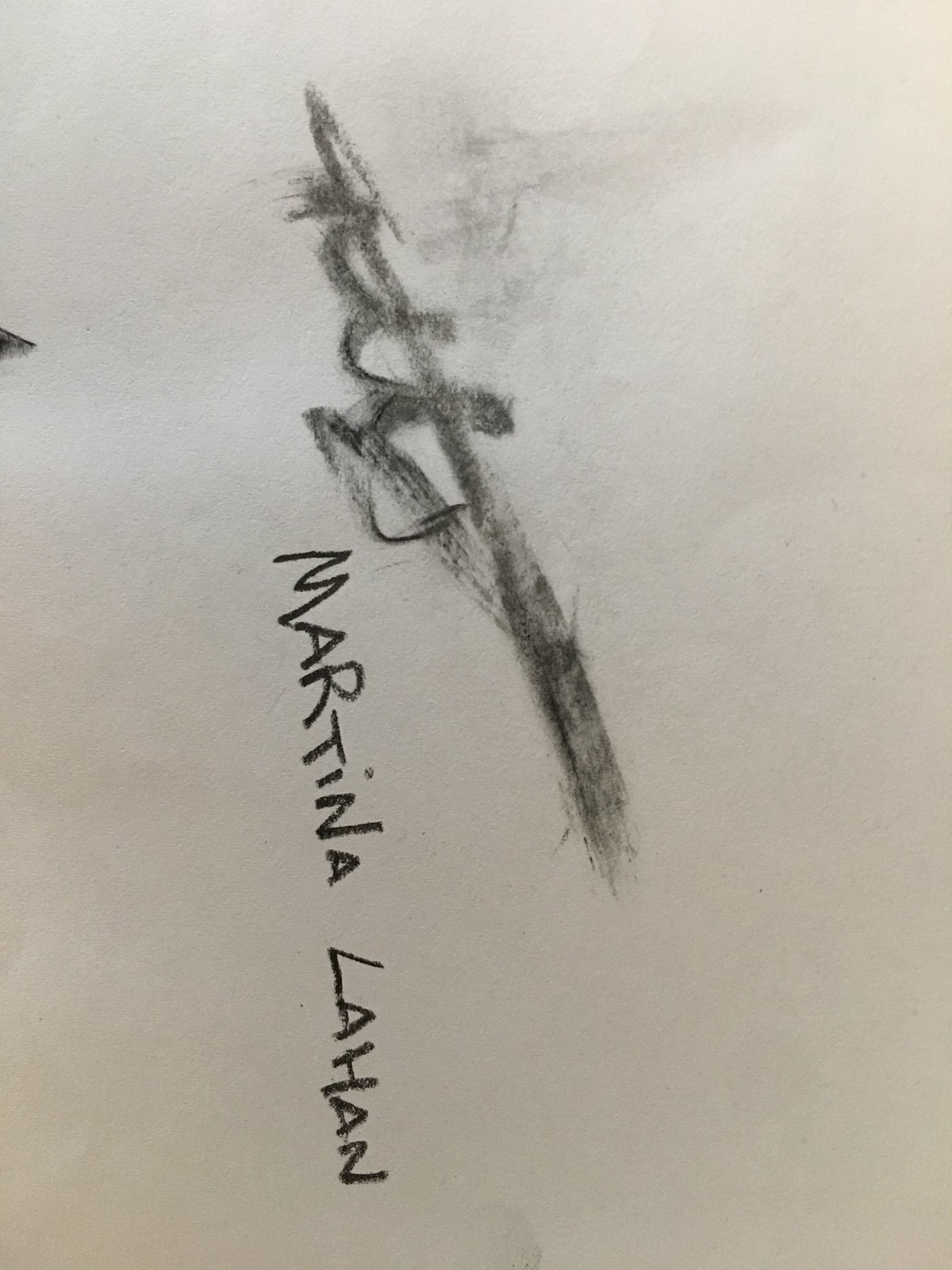The image features a piece of artist-quality sketch pad paper. In the center of the paper, the name "Martina Lahan" is handwritten, with each letter artfully inscribed to read "L-A-H-A-N." Below this name, the artist used charcoal to create an abstract design that begins with a prominent line resembling the letter "J," gracefully curving downwards and then back up. Interspersed around this main line are various squiggles and unstructured markings, suggesting a freeform, experimental sketch. The charcoal work includes notable smudging, indicative of the artist's hands-on approach and the medium's inherent messiness. This image appears to be a snapshot from Martina Lahan's sketchbook, capturing a moment of spontaneous artistic expression without depicting any concrete, recognizable forms.